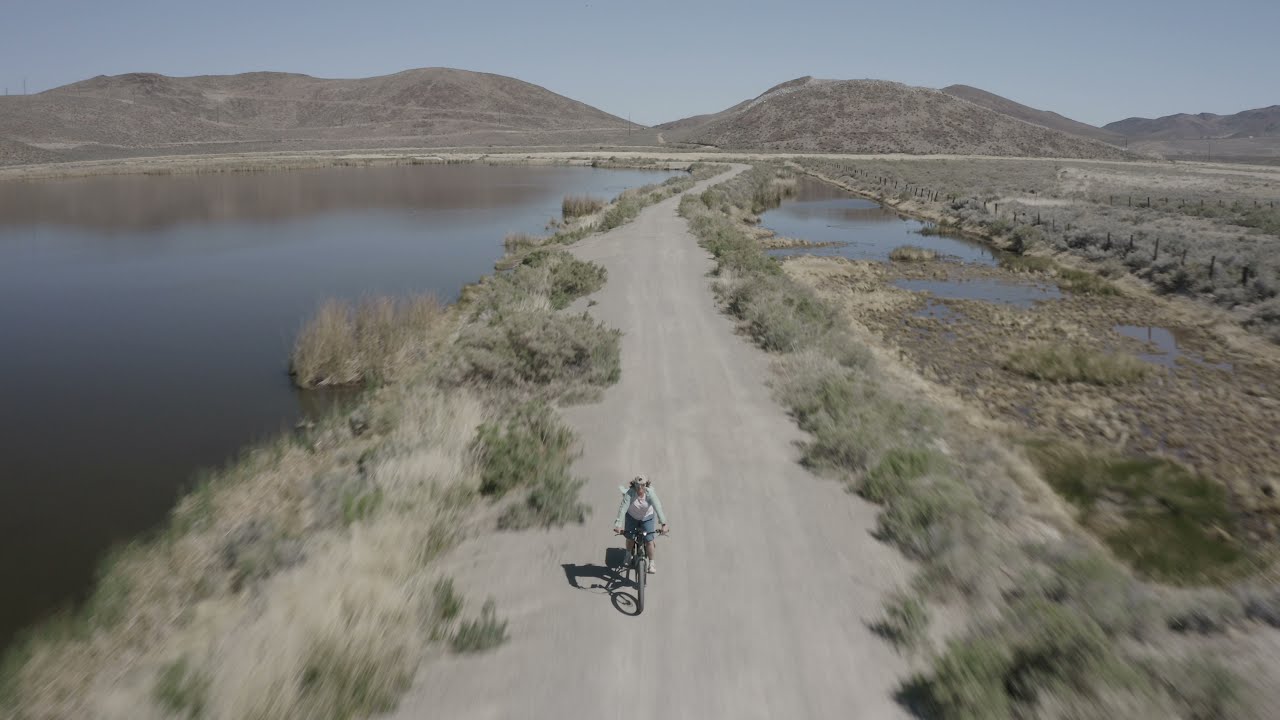This high-angle drone shot, taken from approximately 15-20 feet above the ground, captures a woman bicycling on a tan dirt road. She is looking up at the drone and wearing a green long-sleeve shirt over what appears to be a pink shirt, blue shorts, and a tan or green hat. The dirt road stretches directly beneath her and separates two distinct bodies of water: on the left, a larger lake with tall, beach-like grasses; on the right, a smaller pond-like strip possibly formed by overflow or high tide, with a wooden fence and what seems to be farmland beyond it. The background reveals a dry, mostly barren landscape with brown and tan hills, devoid of lush vegetation, emphasizing the desert-like environment under a sunny sky.